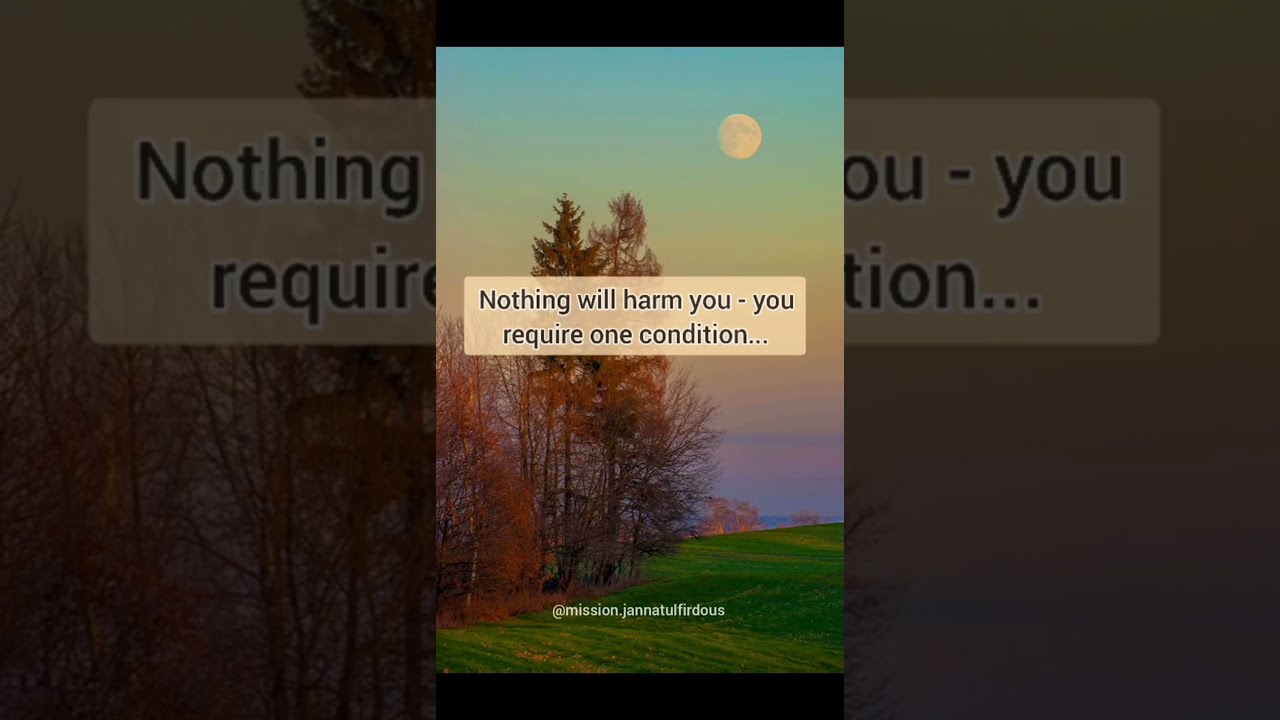The image depicts a wide, vivid grassy hillside with sparse, very tall, brown trees on the left, many of which are bare or have brown and golden leaves that have mostly fallen off. The hill gradually slopes down into what appears to be an ocean or a lake in the distance. The sky, suggesting either sunset or dawn, displays a beautiful gradient transitioning from blue to red, yellow, orange, and turquoise, with a white moon visible. The central feature of the image is text that reads, "nothing will harm you, you require one condition," accompanied by a user handle at the bottom. The photograph is taken vertically, and its background, a faded version of the same scenic landscape, adds depth to the scene.